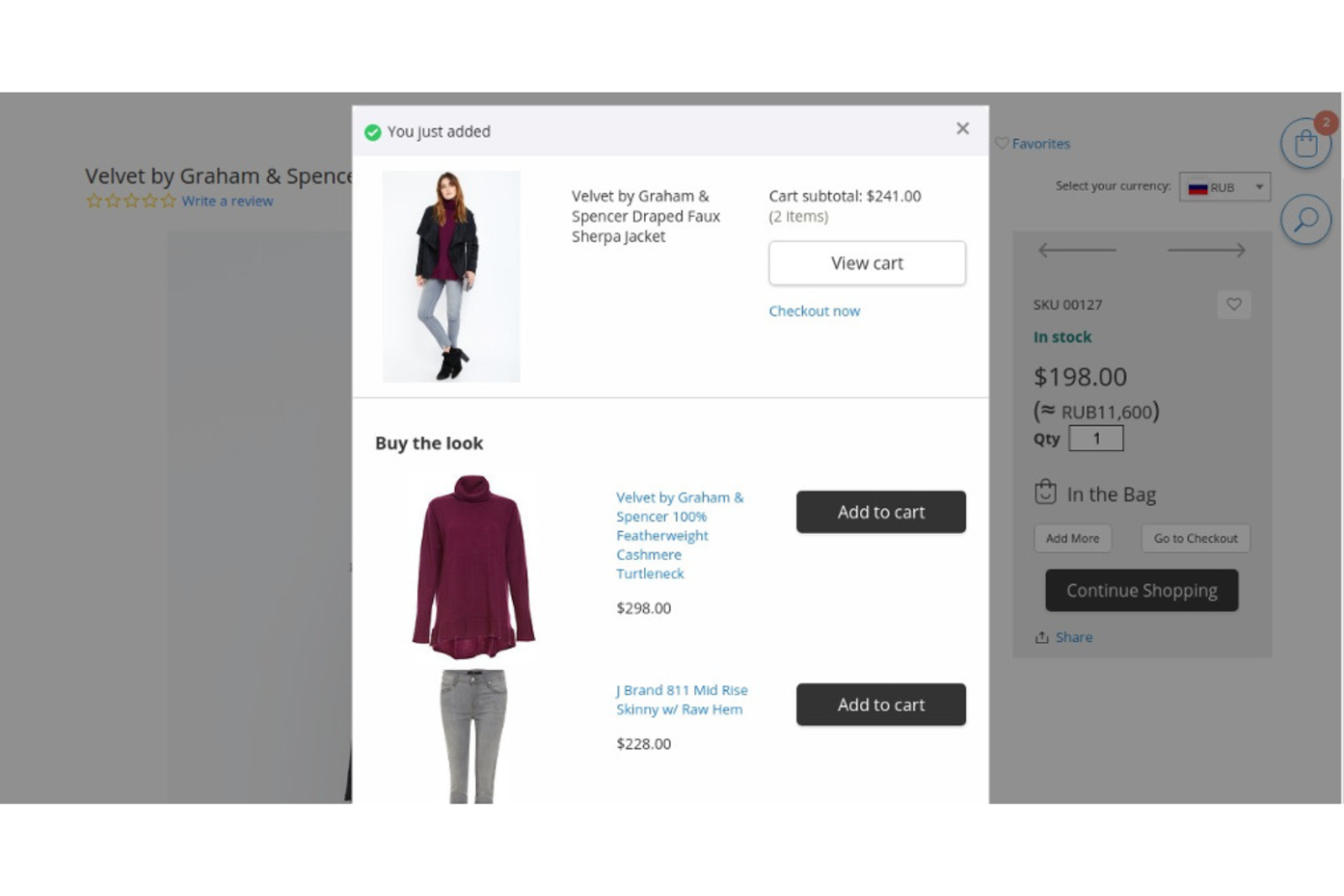The image depicts an individual in the process of online shopping at a clothing store. At the center of the image, a pop-up box appears, indicating that the shopper has just added an item to their cart. In the top left corner of this pop-up, there is an image of a woman modeling the clothing item. She is wearing a black jacket, a maroon shirt, light blue jeans, and black heels. The model has fair skin and brunette hair.

To the right of the model's image, there is a detailed description of the product: "Velvet by Graham & Spencer Draped Fox Sherpa Jacket." To the right of the product name, the cart subtotal is listed as $241. Beneath the subtotal, it notes that there are two items in the cart, with an option to "View Cart" in a rectangular box and a "Checkout Now" link displayed in blue text.

In the top left corner of the pop-up, the words "You Just Added" are prominently displayed alongside a green checkmark. In the lower half of the pop-up, there is a section labeled "Buy the Look," which provides links to the top and bottoms that the model is wearing. Additionally, in the background on the far right side of the image, the price of the black jacket is visible, listed at $198.